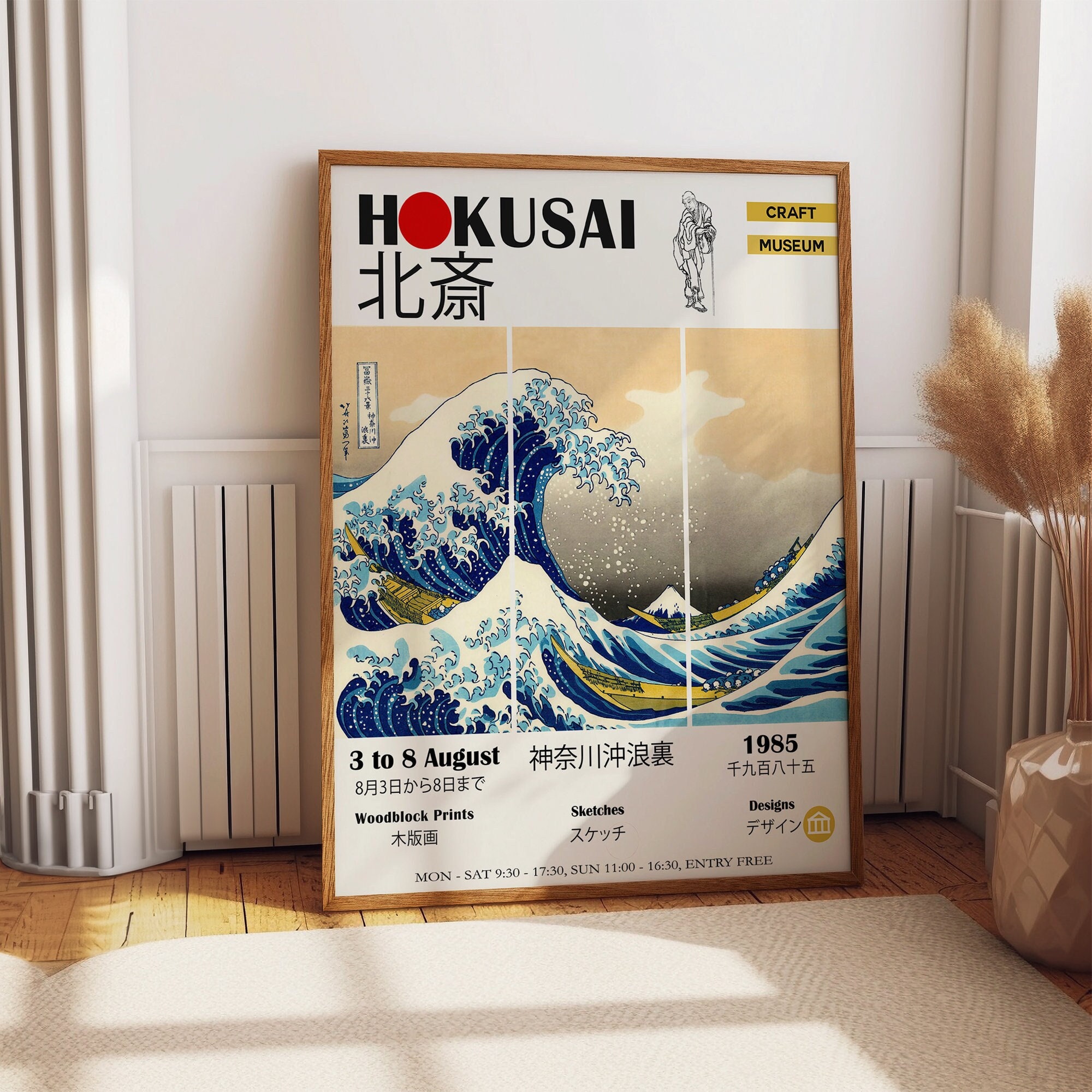In a simplistic and somewhat stark room with cream-colored walls and a light oak plank flooring partially covered by a white rug, stands a framed poster leaning against the wall. The focal point of the scene, the poster, advertises an exhibit at the Craft Museum held from August 3rd to 8th, 1985, showcasing woodblock prints, sketches, and designs. Written in both English and what appears to be Japanese, the top of the poster prominently features the word "HOKUSAI," highlighting the famous artwork of a stylized ocean wave with cresting navy blue and white-tipped waters. Above the waves, almost ethereal, is the image of a spiritual figure with arms outstretched. The wooden frame of the poster harmonizes with the light oak flooring, adding to the room's minimalistic decor. A large vase in the right corner of the room holds a stem with a fluffy top, closely resembling a cream-colored rug, enhancing the serene atmosphere of the space.